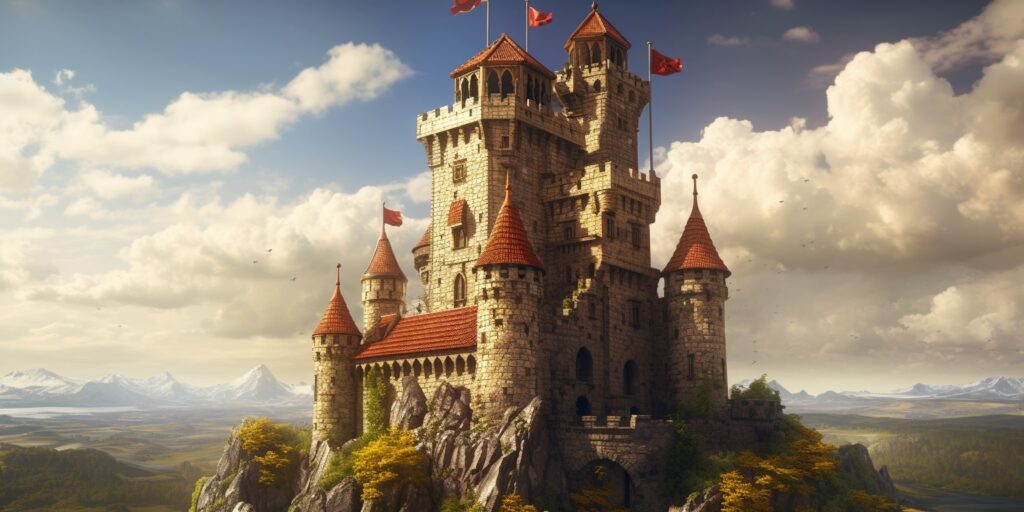This horizontal, computer-animated image showcases a medieval-style fantasy castle perched dramatically on a cliff or mountain, with a stunning landscape setting. The castle, constructed from gray stone with patches of moss, features a series of distinct rounded and blocky towers topped with red terracotta-style roofing. The central towers prominently display red flags fluttering atop. In the background, a serene valley extends, surrounded by gentle hills and towering snow-covered mountains under a partly cloudy sky, where fluffy white clouds contrast against patches of vibrant blue. The lighting suggests a sunny day, with cloud shadows adding depth to the scene. The castle, with its intricately designed stonework and multiple towers, including a front-facing balcony, evokes an enchanting fantasy atmosphere, reminiscent of settings from storybooks, movies, or video games.